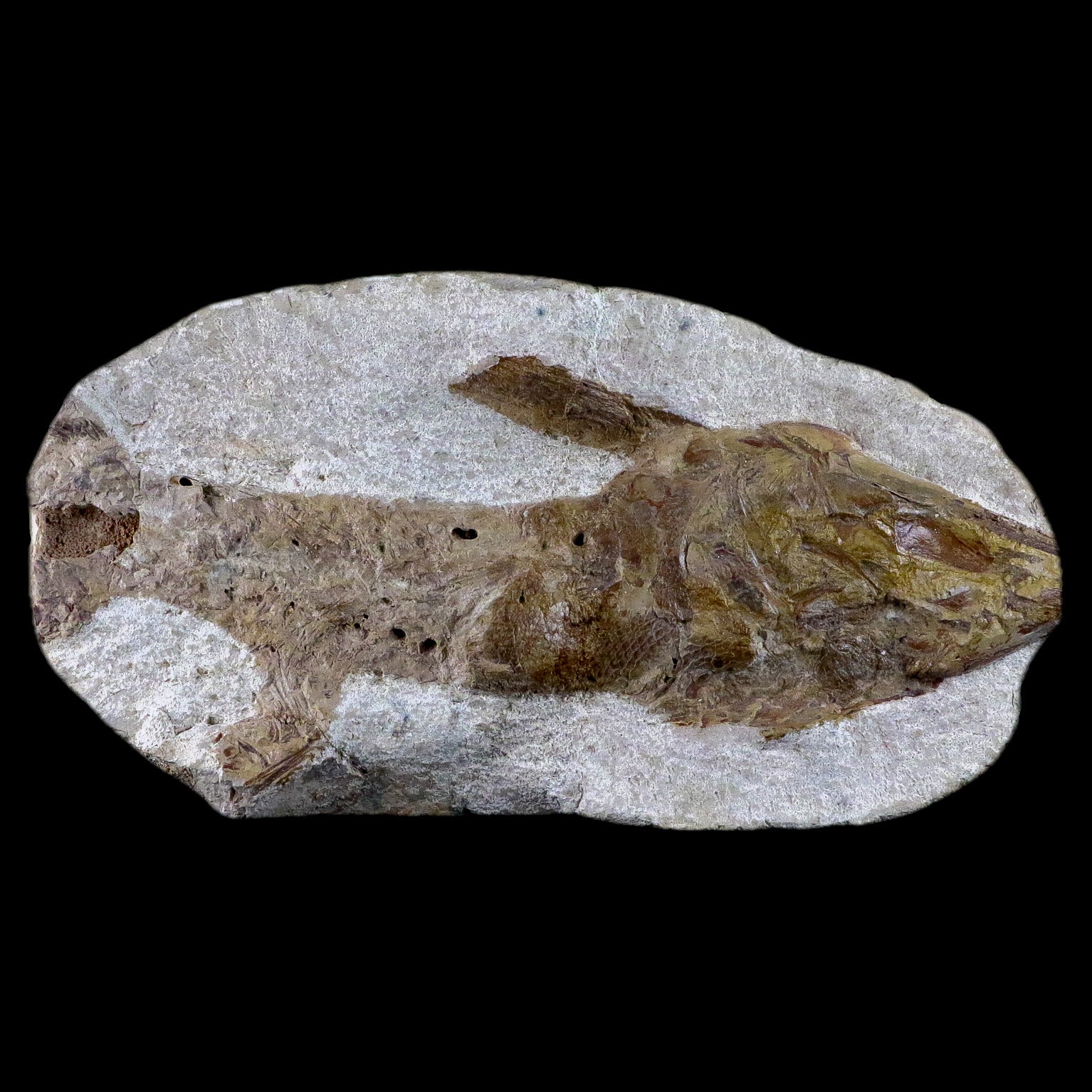The photograph captures an ancient fish fossil embedded in a light stone against a solid black background. This setting allows the fossil to stand out prominently. The fossil is partially protruding from the stone, with the front half more distinctly preserved, displaying a dark greenish tone, while the back half is more of an imprint. Detailed examination reveals notable features such as the fish’s tail fin, lower fin, and top fin, clearly indicating its identity. The fossil’s coloration varies from yellowish brown to dark green, and some parts exhibit scale-like textures, adding to the sense of antiquity and preservation. The stone itself shows grey calcification contrasting against the fossil’s distinct hues, emphasizing the fossil's organic details against the sterile background.